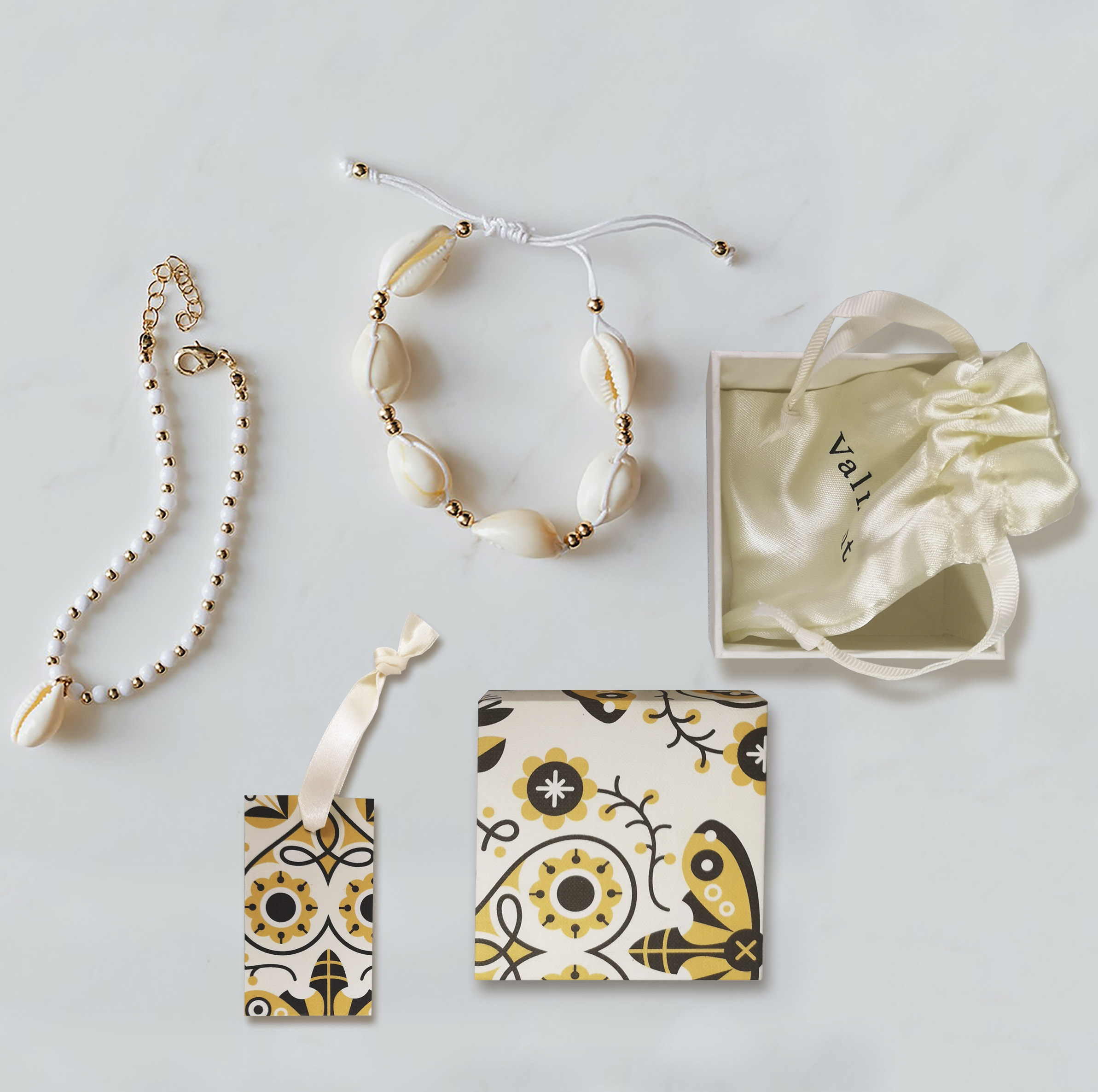In this detailed photo likely intended for a catalog or advertisement, five items of jewelry and packaging are meticulously arranged on a white background. Starting from the left, there is a beaded bracelet featuring an alternating pattern of white and gold beads, with a white seashell pendant prominently at its center and secured by a gold-colored clasp and chain. Next to it is another bracelet made of several white seashells interspersed with gold beads, strung on a white pull-string with two beads at its ends. Accompanying the jewelry is a cream-colored satin gift bag with cinch ties, emblazoned with a partially visible brand name starting with "V-A-L-L." Adjacent to it is a coordinated gift box adorned with a sophisticated yellow, black, and cream floral design, matching an additional small luggage or gift tag tied with a satin ribbon, completing this elegant presentation.